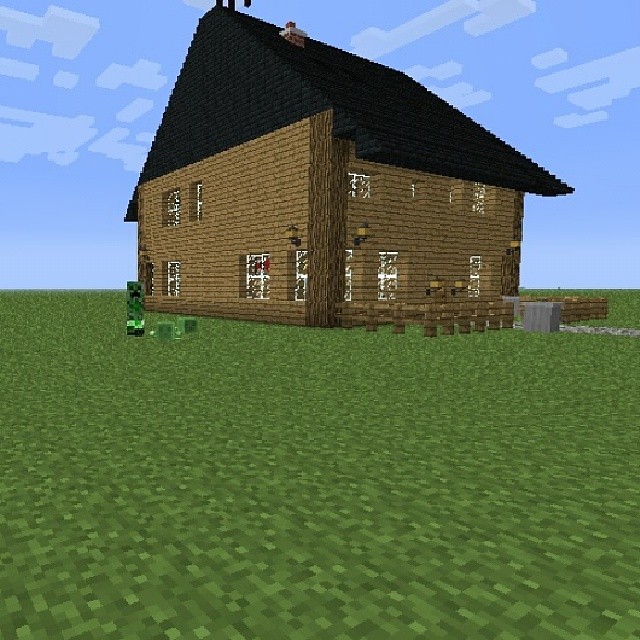The image showcases a meticulously constructed house within the popular video game, Minecraft. The house features a striking black triangle roof that slightly overhangs the wooden structure beneath it. The building itself is square in shape and is crafted from two types of wood. The corners are accented with unstripped logs, rich with bark, contrasting vividly with the lighter, stripped wooden planks that make up the walls. This attention to material detail adds a rustic charm to the house.
 
The house is well-lit with various light sources positioned around its exterior, including the sides and front, enhancing its inviting appearance. Prominent glass windows punctuate the wooden walls, allowing light to flood the interior. Adjacent to the house, a notable character from the game, a Creeper, stands menacingly to the left side of the structure.

The backdrop features a serene, clear blue sky adorned with a few scattered clouds, casting soft light over the flat, expansive landscape surrounding the house. Adding to the homely appeal, a stone chimney rises from the roof, suggesting the presence of a cozy fireplace inside. This well-crafted house epitomizes the creativity and endless possibilities within the Minecraft world.